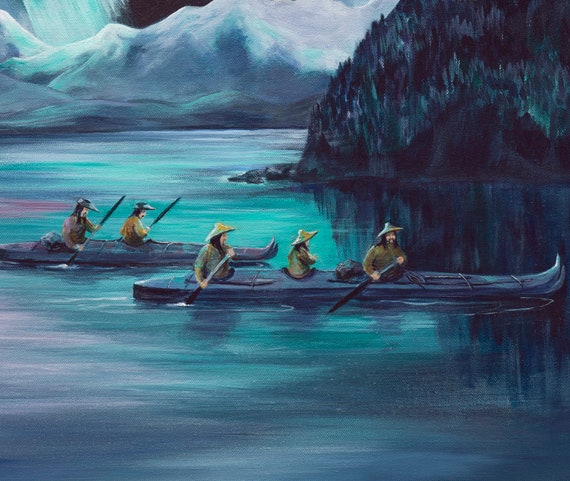This painting depicts a serene and picturesque scene featuring two grayish canoes on a vibrant waterway awash with an array of colors including blues, pinks, purples, turquoise, and dark blues. The canoes are elongated with front ends that curve upward toward the sky, creating a sense of movement and elegance. In the first canoe, three men with distinctive long black hair and long mustaches, dressed in hats reminiscent of Asian culture, are seen rowing. One of them, possibly a female or child, is seated between two paddlers. The hats in this canoe are tan with white brims. In the second canoe, two men are rowing, both also wearing traditional hats though theirs are darker with a larger front brim. The closed-top canoes suggest the people's legs are not visible, emphasizing their traditional attire and engaged rowing action. The background is dominated by majestic mountains, a mix of snow-covered peaks and lush green hills. Additionally, the upper right-hand corner features a dense, dark green wooded area, enhancing the natural beauty and calmness of the scene. The men appear to be aiming for a distant shore, immersed in their tranquil journey.